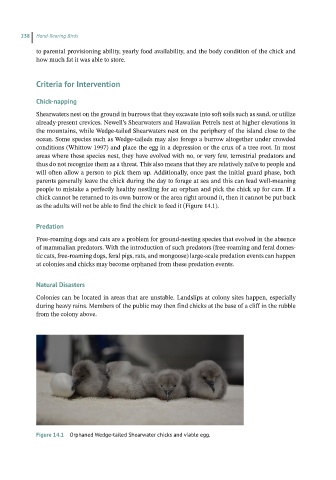This image depicts a page from what appears to be a textbook or guide about caring for hatchling birds. The page is numbered 238 and contains multiple sections of text, though the specific chapter heading is unreadable. The text seems to discuss topics such as "Criteria for Intervention," with subtopics including "Chick Napping," "Predation," and "Natural Disasters." A partial sentence visible on the page talks about factors like "parental provisioning ability, yearly food availability, and the body condition of the chick." The headings are highlighted in teal color. At the bottom of the page, there is a black and white photograph featuring four very young, fuzzy, gray chicks with small dark gray beaks, resting on a soft white surface. To the left of the chicks lies a viable egg. The caption under this photograph reads, "Figure 14.1, Orphaned Wedge [...] Chicks and Viable Egg," although some text remains unclear.